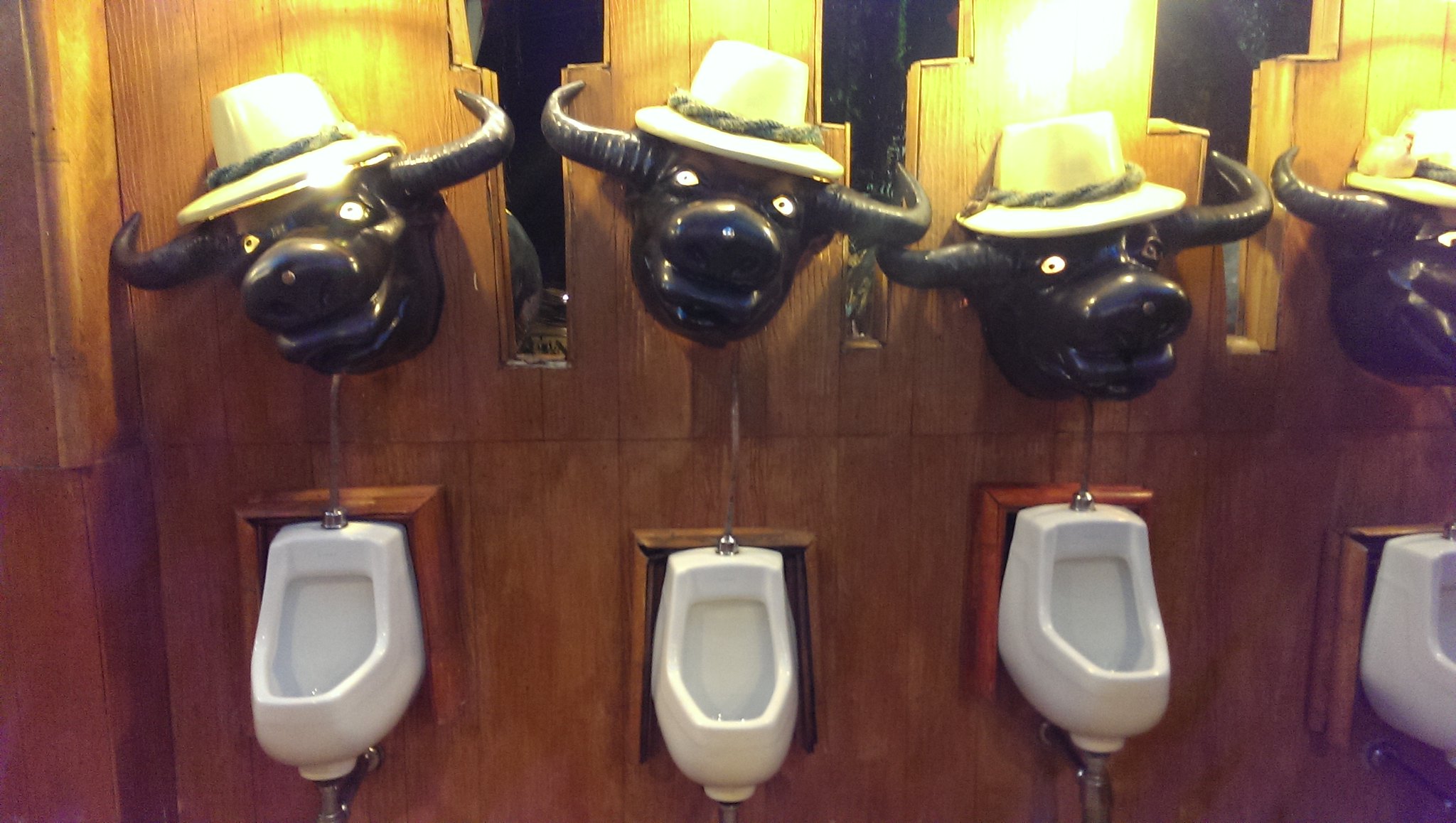This color photograph captures the inside of a men's public restroom, drawing attention to its unique and whimsical decor. The medium wood-colored wall serves as a backdrop for four white porcelain urinals, each set within a small indentation in the wall. Above each urinal, there is a black bull's head sculpture. These cartoonish, roundish bull heads feature black horns curving backward and are adorned with tan, wide-brimmed hats decorated with strings. The bulls' heads also have white eyes with pin-prick pupils, adding a quirky touch to the scene. The restroom is devoid of people, real animals, or any written signage, focusing solely on this unusual and amusing display.